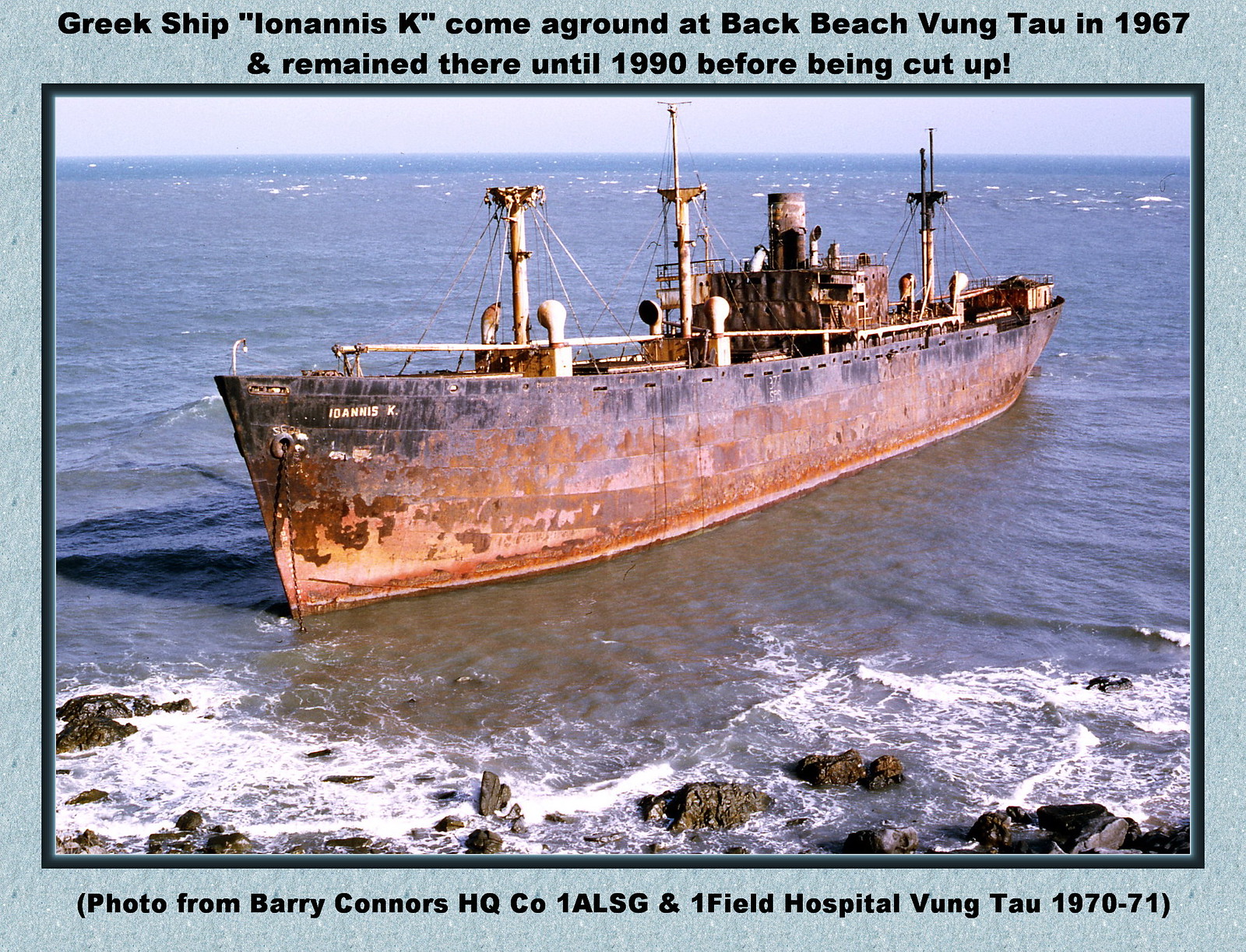This large square image, reminiscent of a postcard and bordered in light blue, prominently features a weathered, rusted cargo ship, named Ionis K, stranded near the shore. The ship appears grey and brown with varying shades of rust. Visible in the foreground are large rocks, with rough greyish-blue ocean waters splashing against them. The vessel is positioned diagonally in the center of the image, with the expansive sea as its backdrop and a faint sky above.

Caption details are included in bold black letters at both the top and bottom of the image. The top reads: "Greek ship (Ionis K) came aground at Back Beach, Vung Tau in 1967 and remained there until 1990 before being cut up." The bottom caption notes: "Photo from Barry Connors, HQ Company, 1ALSG, and One Field Hospital, Vung Tau, 1970-1971." The setting is likely Vung Tau, Vietnam, given the historical context.